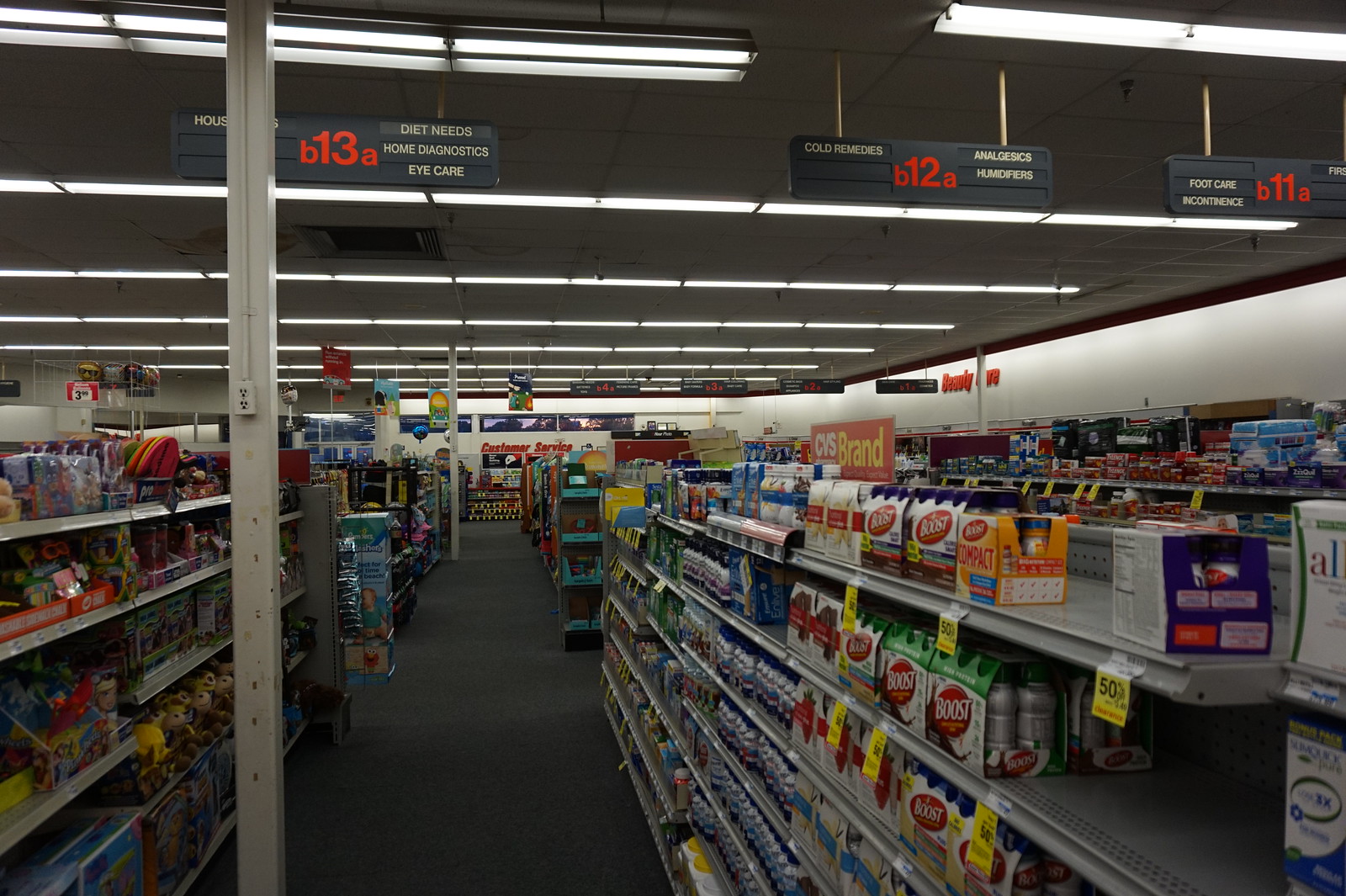The image captures the interior of a well-lit CVS store, specifically looking down aisle B13A, which is designated for diet needs, home diagnostics, and eye care. The overhead fluorescent lights illuminate various shelves stocked with products on both sides of the aisle. Visible signs also indicate the presence of aisles 12B and 12A offering cold medicines, analgesics, and possibly humidifiers, as well as aisles 11B and 11A dedicated to foot care and incontinence items. Some shelves feature products like Boost Nutritional Supplements and other dietary items, with yellow sale tags prominently displayed under them. The store is characterized by a neat, off-white interior, reminiscent of a typical CVS layout.